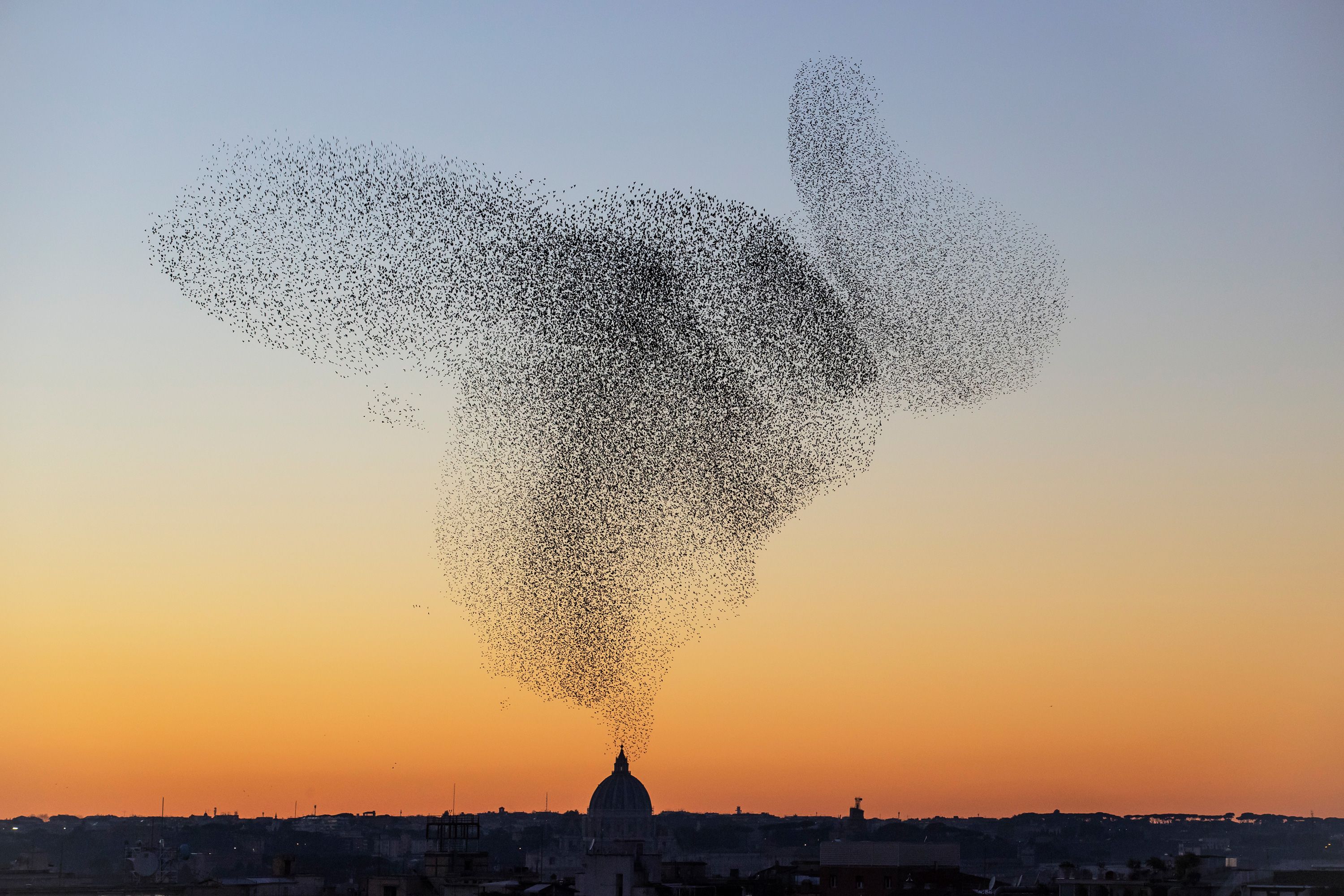This photograph captures a striking sunset or sunrise scene, horizontally aligned, with a gradient sky that transitions from a deep orange at the horizon to a gentle blue at the top. Dominating the bottom 20th of the image, a darkened band of land silhouettes against the vibrant sky. Central to this landscape is a dome-like structure, possibly a temple or tower, topped with a narrower spire. This building stands about a centimeter tall and wide, and it's flanked by a smaller, similar structure to the right.

The photo’s main focus is an impressive formation of birds, which creates a dense, pointillist pattern in the sky. This flock of black birds resembles a brain shape when viewed from a distance, with two round, floppy, dog-ear shapes on either side. The overall formation creates the illusion of drifting smoke due to the clustered arrangement of birds, appearing darker where the birds are densely packed and lighter where they are sparse.

Scattered lights from buildings below punctuate the dark land, while the dome's silhouette adds a touch of architectural grandeur to the scene. The image, likely taken by a skilled photographer, captures a beautiful and somewhat surreal moment of nature converging with human-made structures.